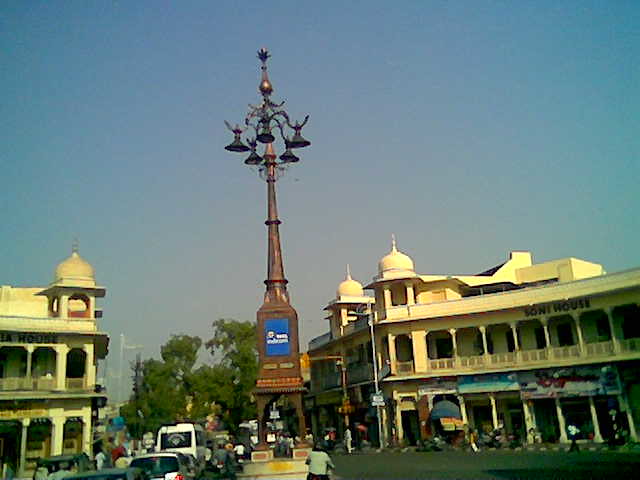This detailed image captures a bustling town scene with intricate elements. Taken from the passenger side of a car amidst noticeable traffic, a prominent bronze structure dominates the center of the image, intricately designed with curved arms holding five bell-shaped lanterns, and topped with a bulbous crown. This central light post, supported by a four-stand base, also features a blue sign with unreadable text.

Surrounding the roundabout, on both the left and right sides of the street, are two-story buildings, yellow in color, displaying signs that partially read "Sony house." These buildings feature balconies with gated posts and small spires or domes on top. The street is lined with various shops, and the sidewalks teem with people walking.

A blue-tented food cart occupies a corner of the street. Numerous vehicles, including vans, motorcycles, scooters, cars, and a white bus, navigate the roads beneath a sky that transitions from blue to white towards the center. Green trees add a touch of nature to this urban environment, which is covered in a mix of cement and blacktop paving. The entire scene encapsulates the lively and detailed atmosphere of a bustling town center.